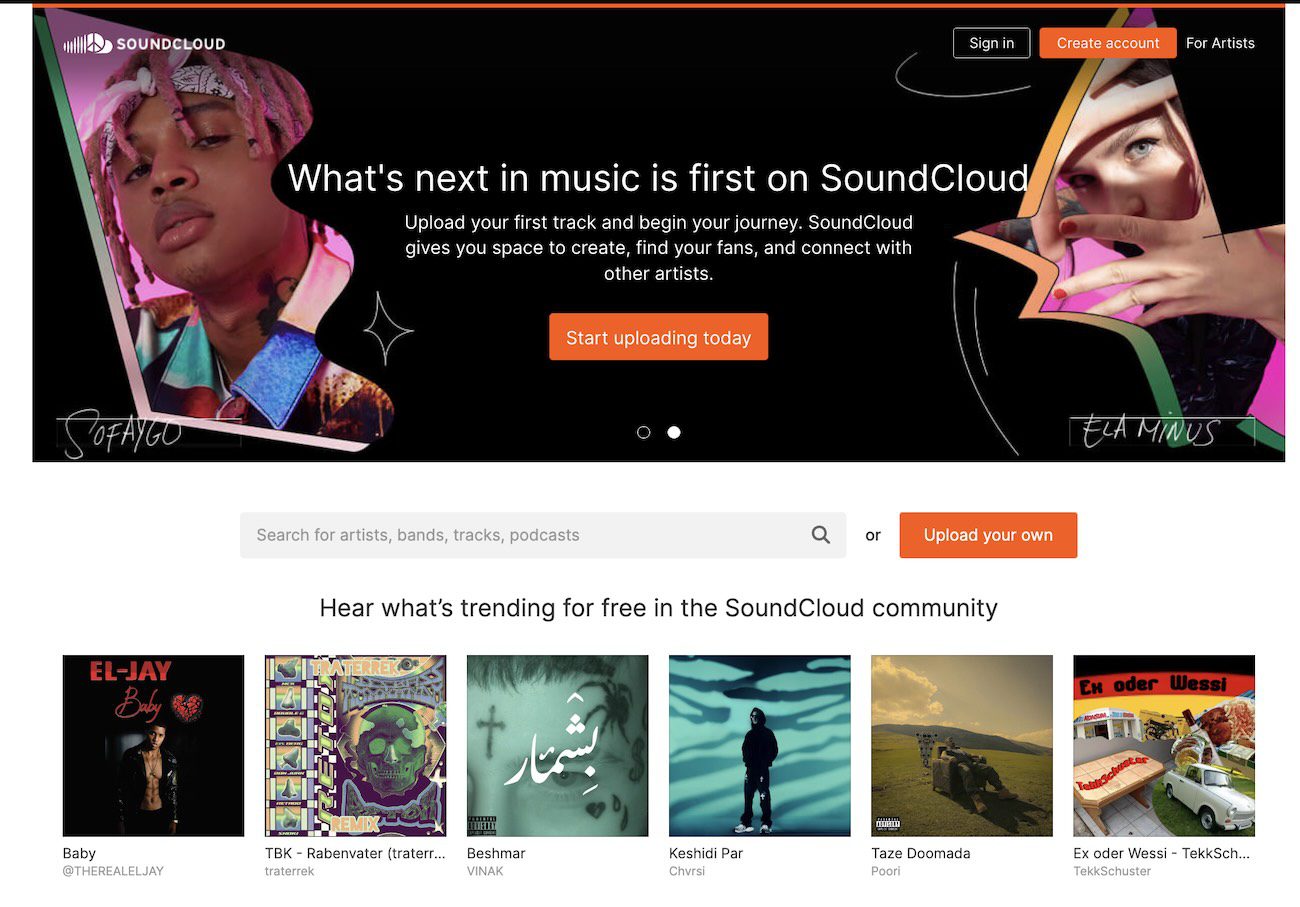The image displays a sleek black rectangular banner at the top. On the upper left side, it features the SoundCloud logo accompanied by a sound wave icon and a peace sign. On the upper right side, there are two buttons: a black "Sign In" button and an orange "Create Account" button. The banner emphasizes SoundCloud as a platform designed for artists.

Below the banner, the image showcases two individuals. On the left, there is a black person with distinctive pink braids that fall past their eyes and what appears to be a neck tattoo. On the right, a white person with blue eyes and red fingernails is depicted. The caption accompanying these images reads: "What's next in music is first on SoundCloud. Upload your first track and begin your journey. SoundCloud gives you space to create, find your fans, and connect with other artists." Below this text, there's a prominent orange button that says "Start Uploading Today."

At the bottom of the image, a search bar invites users to "Search for artists, bands, tracks, and podcasts," accompanied by another orange button labeled "Upload Your Own."